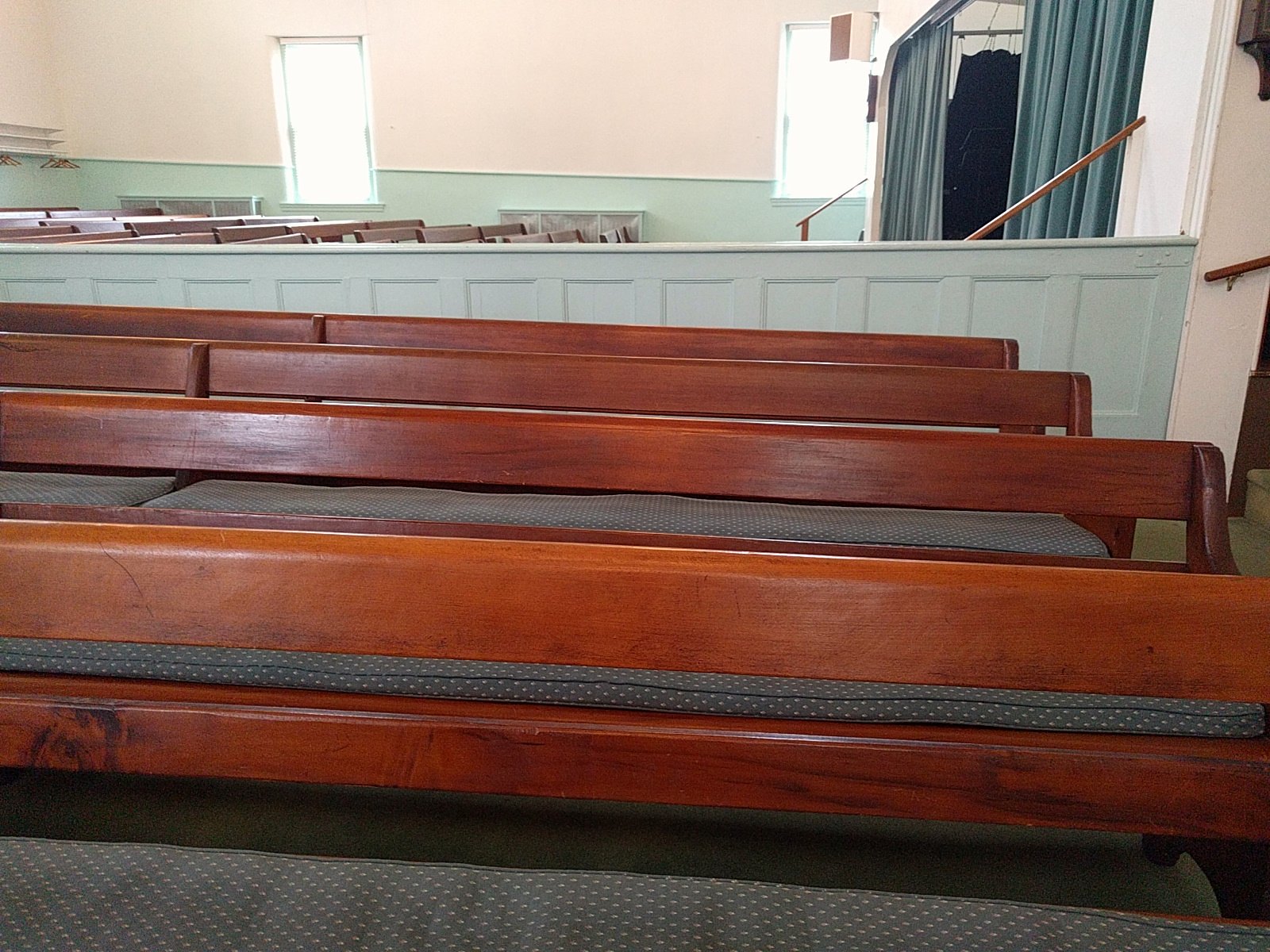The image depicts the interior of a church, featuring a series of long, brown pews with gray fabric seats adorned with cream-colored dots. The photograph is taken from a frontal angle, primarily showcasing the backs of the pews, which are made of dark red-orange wood. The pews are lined up in a carpeted area, with no armrests. In the foreground, four of these pews extend horizontally, partially obscured on the right side.

The background features a light blue-green, or seafoam-colored, half-wall with recessed square patterns. Above this half-wall, the upper section of the wall is painted white. Windows bracket either side of this half-wall, with cutouts and green curtains to the right. Further back, additional pews are visible, oriented to the right, behind the half-wall. On the far right, blue curtains are drawn open, revealing a stage or room with some indistinct, dark mass inside. Adding to the detail, there are handrails and seemingly invisible stairs leading up to this elevated area. The overall scene is bathed in soft, ambient light, giving it the tranquil and reverent atmosphere typical of a church auditorium.